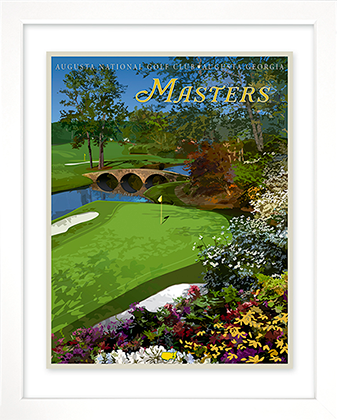This image features a white wooden frame with a white background, presenting what appears to be a beautifully painted magazine cover. Dominating the center is a vibrant scene from Augusta National Golf Club in Augusta, Georgia, identified by the yellow text at the top of the image. At the forefront, a putting green with a yellow flag is visible, casting shadows alongside shadows of nearby trees and flowers, creating a lively interplay of light and shade. Among the lush greenery, there is a sand bunker to the left, and a blue river reflecting the surroundings runs through the middle, crossed by a brown stone bridge with three arches. The bridge leads to more greenery and another flag marking another green zone. The scene is further adorned with an array of flowers in the lower right corner, featuring colors from yellow and red to white and blue, spreading through the upper right portion of the image. Completing the picturesque setting is the word "Masters" inscribed in capital letters in a scripted font, reinforcing the prestigious nature of this golf course scene.